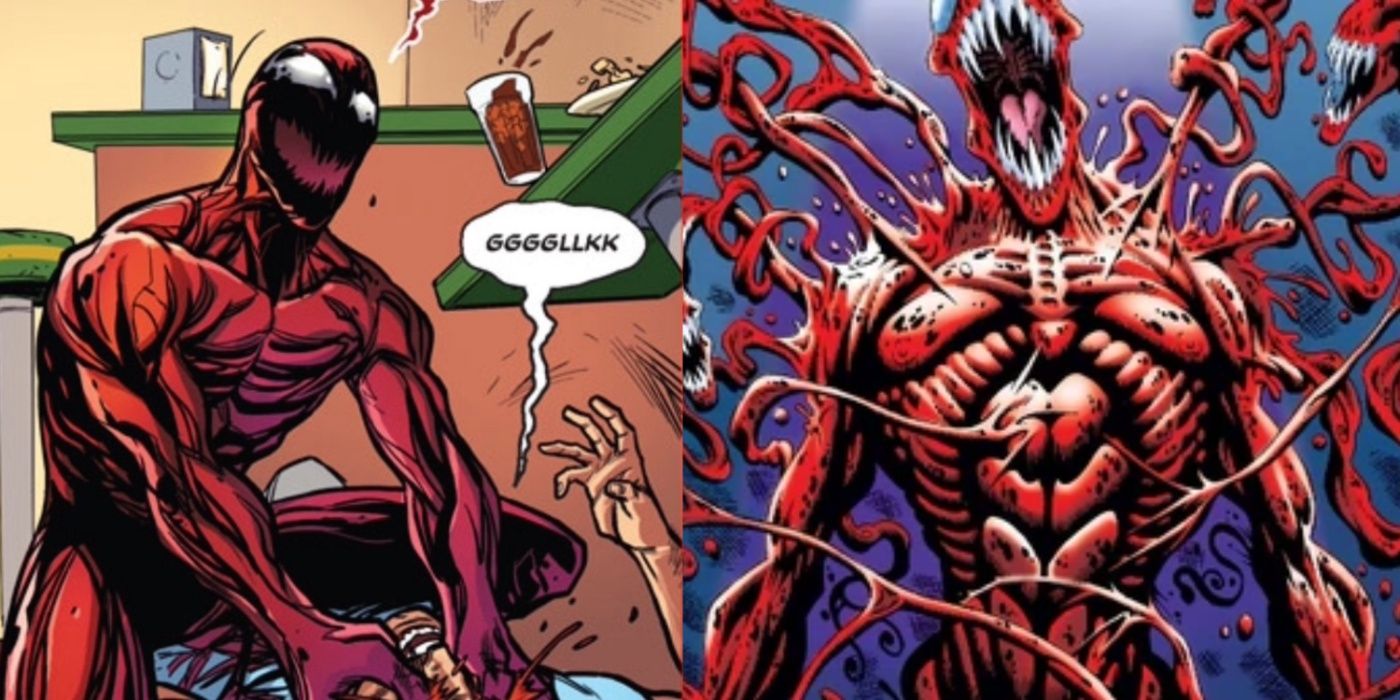In this two-panel comic strip, the left panel depicts the Spider-Man villain Carnage, a red, muscular figure with large, white, squinty eyes, and a wide, sinister smile outlined in black. Carnage is shown crouching over an individual wearing a blue shirt, his left hand choking the victim who lies on the ground. Emerging from the victim is a dialogue bubble that reads "GGGGLLKK". The chaotic scene includes a green table tipping over, spilling a glass of brown liquid with visible ice cubes. In the background, a green bar with a silver napkin holder and white napkins further lines the setting.

In the right panel, Carnage is featured in a more monstrous form, his mouth agape revealing sharp white teeth and a pink tongue. Red flesh and blood-like tendrils are flying off his body, accentuating his fierce transformation. The background is splashed with intense purple and pink hues, heightening the dramatic and violent atmosphere of the scene. Additionally, smaller images of similarly horrifying faces hover around him, emphasizing his terrifying rage.